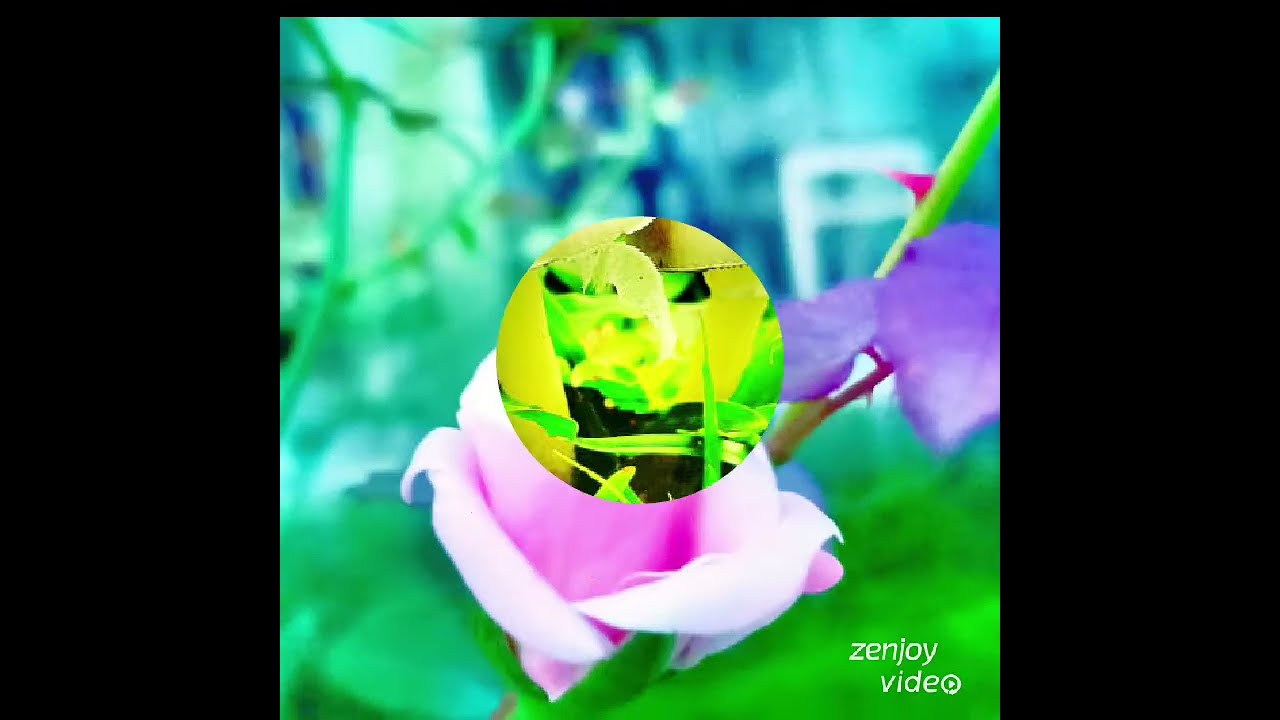The image depicts a man at an outdoor location, possibly a beach, lake, or shallow creek, crouching on a pile of rocks. In the background, a gray, cloudy sky looms over the scene, hinting at possible inclement weather. A narrow strip of rocky ground is visible behind him, separating greenery from a large area of water that appears to be slightly wavy. The man, who has short black hair, is wearing a blue surgical mask, a blue long-sleeved shirt with buttons undone at the front, and dark-colored sweatpants. He is barefoot and seems to have just dipped his hands into the water, with droplets still falling from them. There are clusters of rocks on both the left-hand side and the lower right-hand corner of the image. Additionally, the photo appears to be a screenshot from a video, as indicated by the black borders on the left and right sides and the text "Zen Joy Video" in the lower right corner. The man also wears a red and white scarf, which adds a touch of color to the otherwise subdued setting.